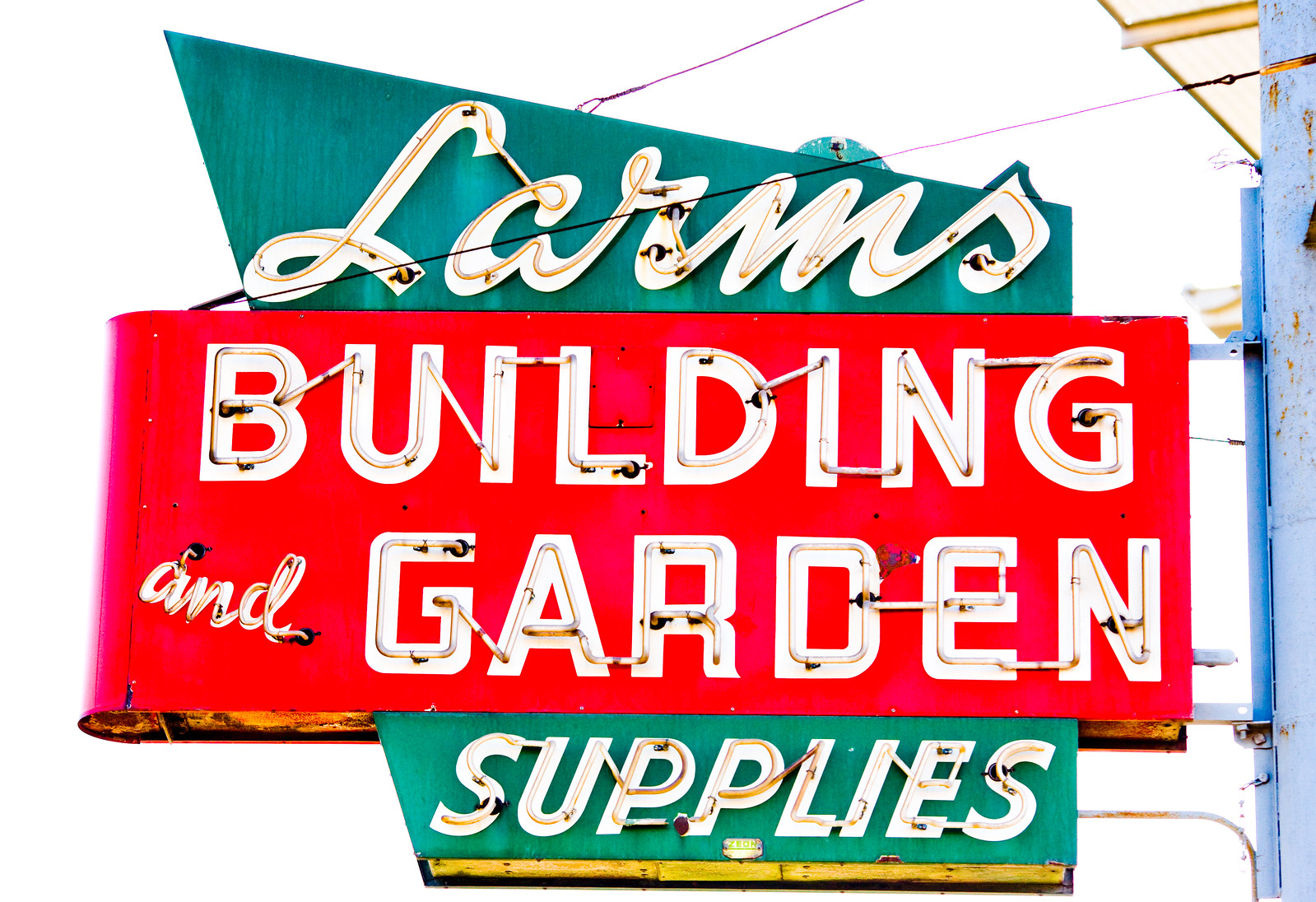This detailed photograph captures a business sign for "Larms Building and Garden Supplies," which is turned off during the day. The sign, hanging horizontally from a vertical blue post, is layered with various colors and shapes that make it visually striking. At the top, "Larms" is elegantly written in white cursive, set against a diagonal dark green background. Below this, a bold red rectangle frames the words "Building and Garden" in white lettering. The bottom section features a green polygonal shape with the word "Supplies" prominently displayed. Embedded within the lettering are neon lights, poised to illuminate the sign with vibrance and visibility once night falls. This intricate and visually layered sign effectively advertises the business while providing both aesthetic appeal and functional readability.